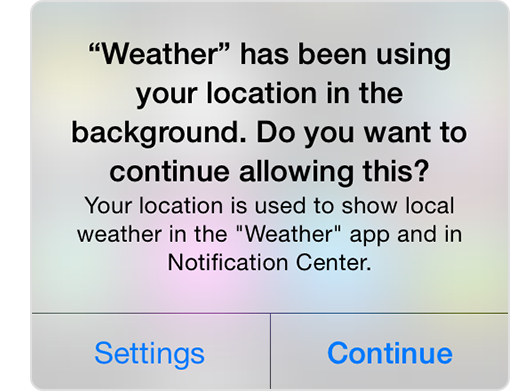This image is a screenshot of a pop-up notification on a mobile device. The notification informs the user about the "Weather" app accessing their location in the background. The message is almost square in shape with slightly rounded edges and features a multicolored, abstract background predominantly in shades of gray, with hints of pink, yellow, and aqua seamlessly blended in. 

At the top, the word "Weather" is displayed in bold and within quotation marks, indicating the name of the app. The message reads, "‘Weather’ has been using your location in the background. Do you want to continue allowing this?" Below this bold text, the notification explains, "Your location is used to show local weather in the Weather app and in Notification Center."

A horizontal gray line separates the message from the options at the bottom. There are two columns–the left column has the word "Settings" in blue, which likely takes the user to the settings menu to modify location permissions for the app. The right column contains the word "Continue," also in blue, allowing the user to maintain the current permissions for the Weather app to access their location. 

Overall, the notification is designed to be a concise and straightforward prompt, ensuring the user is aware of and can manage the Weather app's background use of their location data.